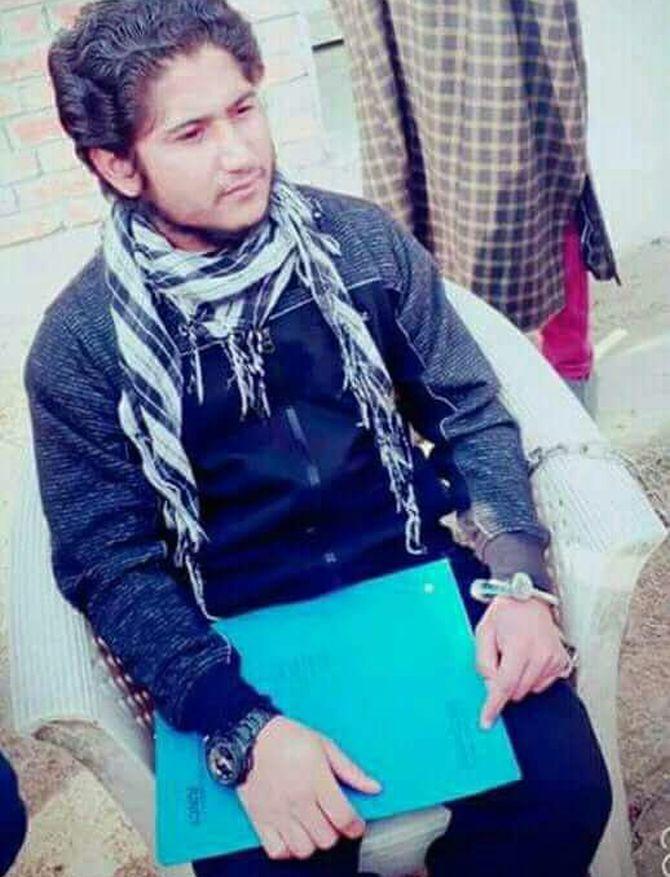The photograph captures a young Caucasian man, likely in his 20s, sitting in a white plastic wicker-style chair outside during the daytime. He is dressed in blue attire, including pants and a zip-up jacket, paired with a white and black scarf wrapped around his neck. His dark, slicked-back hair adds to his neat appearance. The man is holding a turquoise binder close to his lap, clutching it with both hands. He wears a black watch on his right wrist, complemented by a white bracelet on his left wrist. The backdrop features a brick wall and an earthy ground, indicating an outdoor setting. He gazes to his right, and partially visible in the background, a person wearing a poncho and pink pants stands out. The overall scene suggests a chilly season, as inferred from his warm clothing.